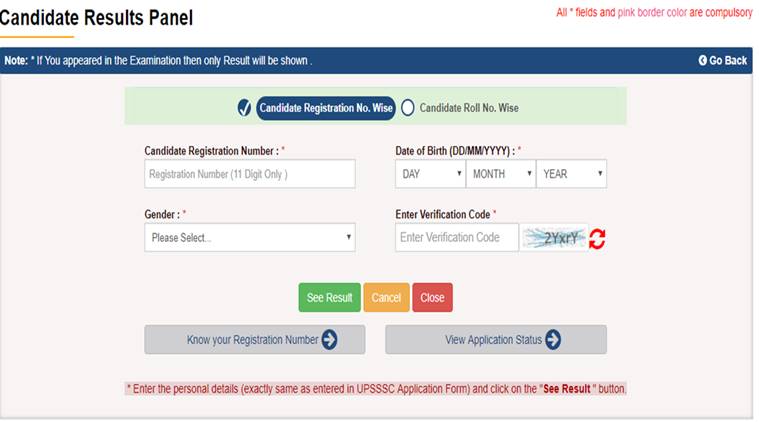The webpage displays a "Candidate Results Panel" at the top in black font, accompanied by a smaller red text message stating, "All fields with pink border color are compulsory." Directly below, a white font on a blue bar provides a notice: "Note: If you appeared in the examination, then only result will be shown," with an accompanying left-pointing arrow, presumably for navigation to the previous page.

The main section of the webpage features a header stating "Candidate Registration No. Wise," next to an actionable button labeled "Candidate Roll Number Wise." Below this are multiple empty text boxes where users can input their candidate registration number, date of birth, gender, and a verification code, prompted by "Enter verification code."

At the bottom of this input section, there are three buttons: a green "See Result" button, a yellow "Cancel" button, and a red "Close" button. Following this, another set of instructions reads, "Know your registration number, View application status," along with a reminder to "Enter personal details exactly same as entered in UPSSSC application form." There is also a smaller red text, "View result," indicating a button for viewing the result.